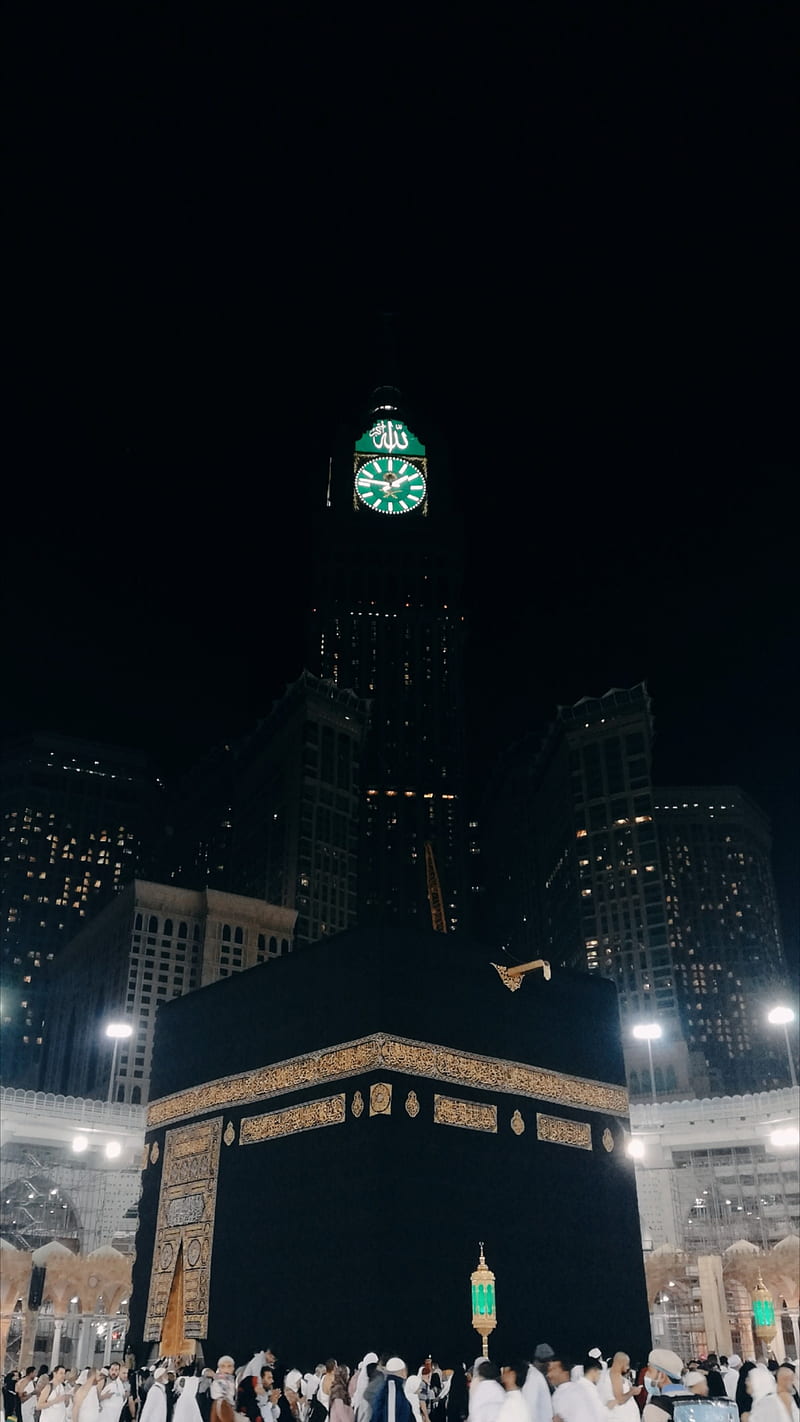This nighttime image captures a bustling scene in what appears to be a city center or courtyard in a Middle Eastern country. The pitch-black sky overhead is devoid of stars, framing a prominent backlit clock tower in the center of the photo. The clock, featuring teal green with white bar markings and Arabic script above it, displays the time as 10 till 2, likely in the morning. Below the clock, the high-rise buildings with tiny, illuminated windows create a dotted backdrop of lights.

In the foreground, a large, square black structure adorned with decorative gold rectangles and a gold band dominates the scene. This structure is surrounded by a throng of people, mostly dressed in flowing white robes, suggesting a form of ceremonial gathering. The area is well-lit, with green and gold lanterns adding to the opulent atmosphere. Despite the crowd's motion, the image captures a significant and possibly cultural event, rich in luxury and tradition.